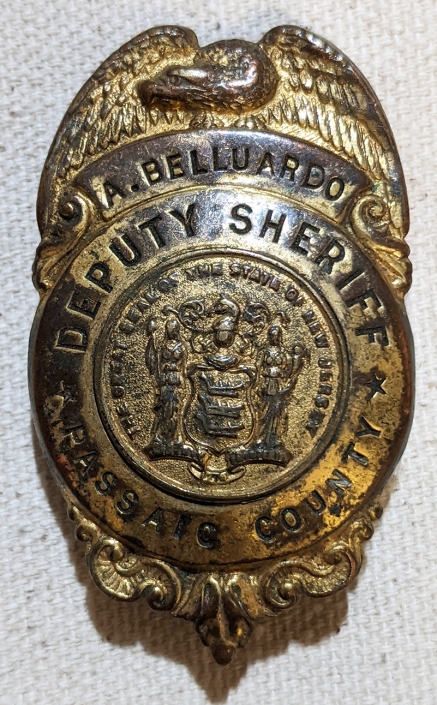This photograph features a discolored deputy sheriff's badge from Pasado County, made of iron with faded gold paint revealing the underlying brownish iron tint. Prominently displayed atop the badge is an eagle with wings spread wide. The badge includes the name "A. Belluardo," indicating it belonged to a former deputy sheriff. The design of the badge also incorporates stars on either side. It is set against a linen cloth background, adding texture to the image.